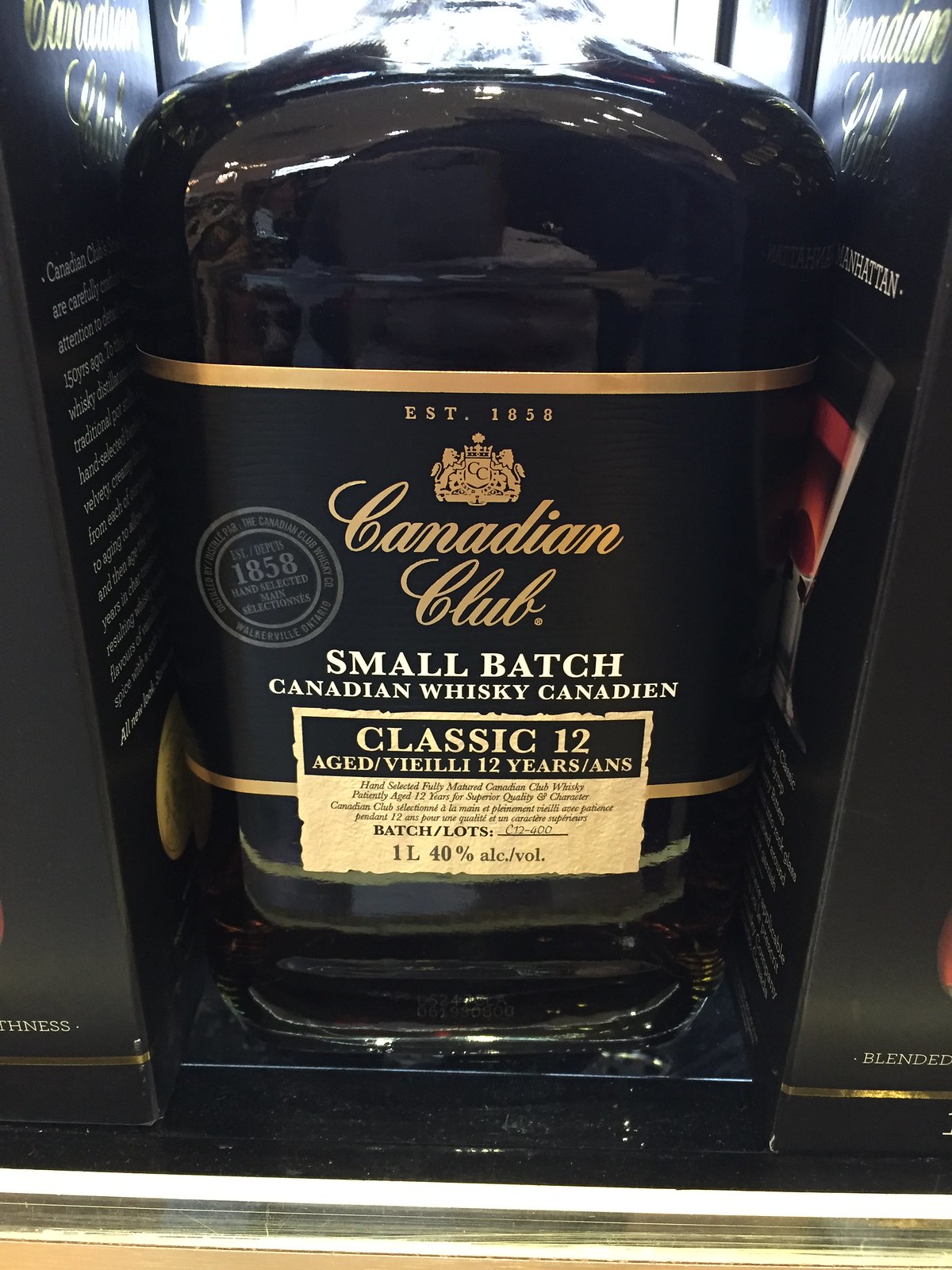The image showcases a tall, rectangular whiskey bottle displayed on a shelf with a gold edge at the bottom. The bottle has a wide, somewhat rectangular shape with a curved top and appears to contain a dark, possibly black liquid. The prominent black label, trimmed with thick gold edges, features the text "EST. 1858" in gold font at the top, accompanied by a gold coat of arms logo with lions on either side. Below this, "Canadian Club" is written in large, cursive gold font, followed by "Small Batch Canadian Whiskey Canadian" in white, all-capital letters. Further down, a large gold rectangle with a black bar reads "Classic 12 Age/Vieilles 12 Years/Ans" in gold text. The bottle is situated between two other boxes, likely of the same whiskey, and is illuminated from above, highlighting its elegant presentation.